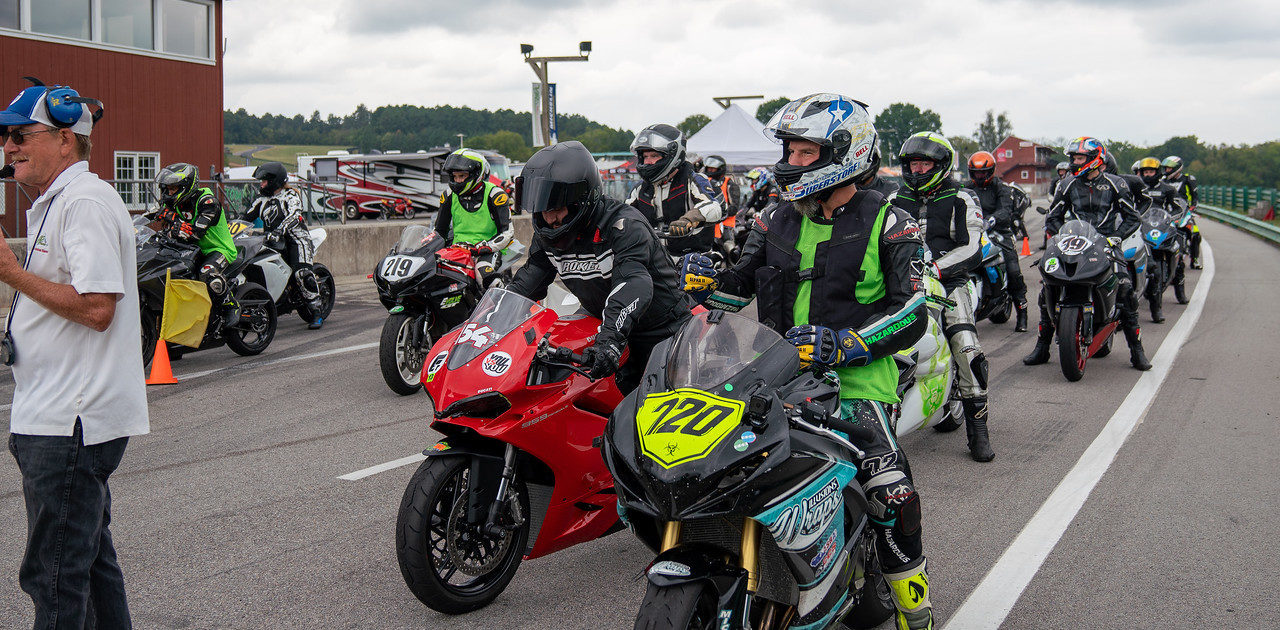On a cloudy day, a photo captures the energetic scene of approximately 20 motorcyclists preparing for a race on a paved street. The riders are assembled in a lineup, each with numbered bikes, suggesting an official racing event. Notable motorcyclists in the foreground include one in a green and black outfit with the number 720 on a black bike, featuring the word "WRAPS" in white on a blue side panel, and another in a black outfit on a red bike with the number 54. Another rider wears a green vest over a black suit and a gray and black helmet, riding a bike marked number 219.

A man in the bottom left corner, dressed in a white shirt, black pants, and a baseball cap, appears to be overseeing the preparations. More riders and enthusiasts can be seen in various positions behind him, all in green, black, and white gear, with notable helmets in orange and red.

The backdrop reveals an overcast sky with gray clouds, a cluster of trees, and a green guardrail extending into the distance. Two two-story red buildings with white window sills stand prominently in the background, possibly serving as central facilities like a clubhouse. Additionally, orange pylons with yellow flags are seen near the track, enhancing the feeling of an organized race event. The overall atmosphere is lively, teeming with anticipation for the race on this late spring or summer day.